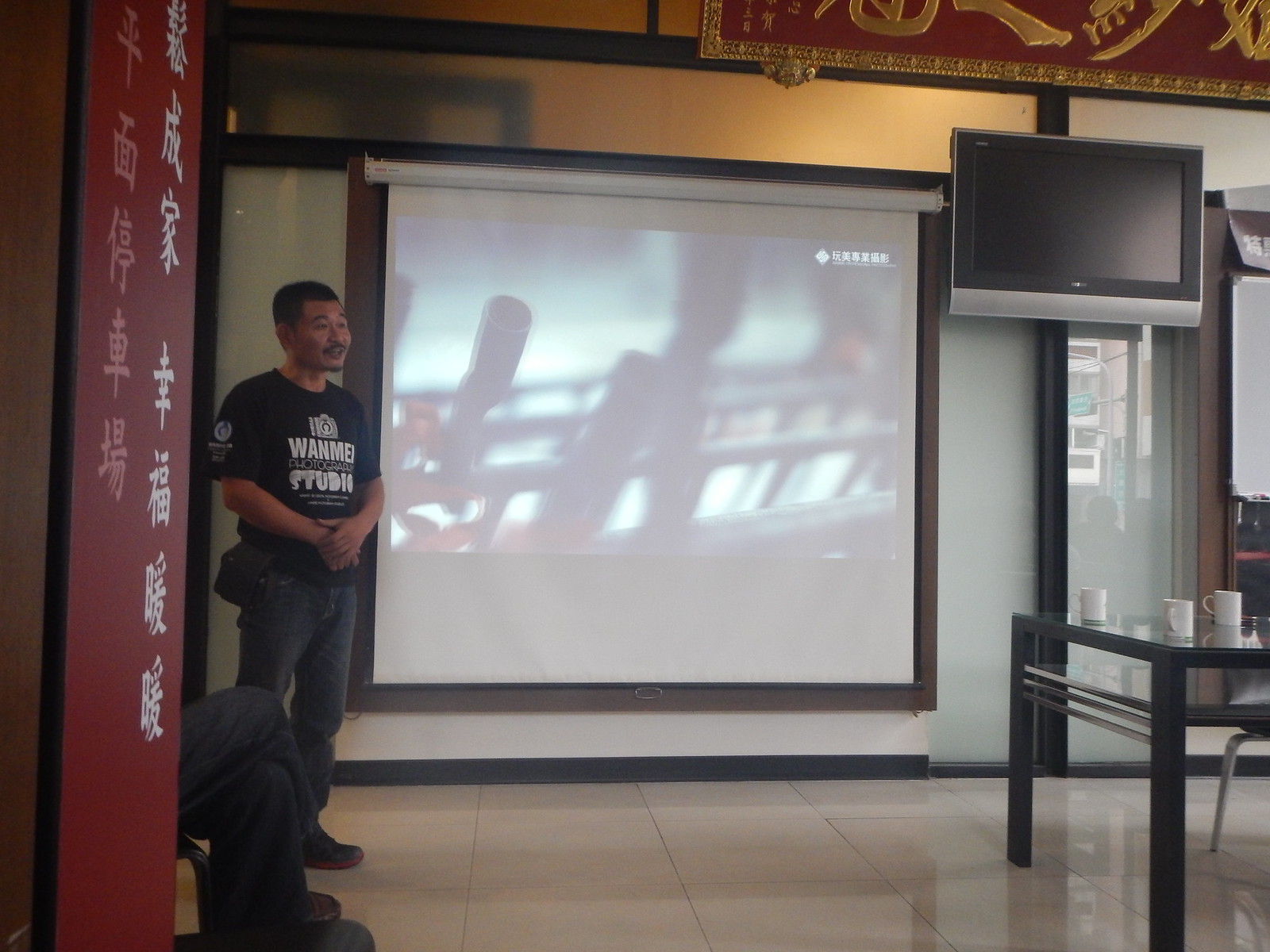The image depicts an Asian man standing in a clean, modern room that features white tiled flooring and a projector screen with indistinct images of metal on it. Positioning himself to the left, the man faces forward and slightly right, dressed in a black t-shirt with white writing and gray pants, his hands held together at his waist. Beside him, to the right, is a white projector screen with a brown border, above which a small, unused television is mounted. Below the TV is a table with three white mugs arranged on it. Dominating the left side of the image, a red banner adorned with Asian characters stretches from the top to the bottom of the frame, partially obscuring another individual seated with legs crossed. The room's modern and tech-savvy aesthetic hints at its use for presentations or meetings, possibly in a Chinese-speaking country.